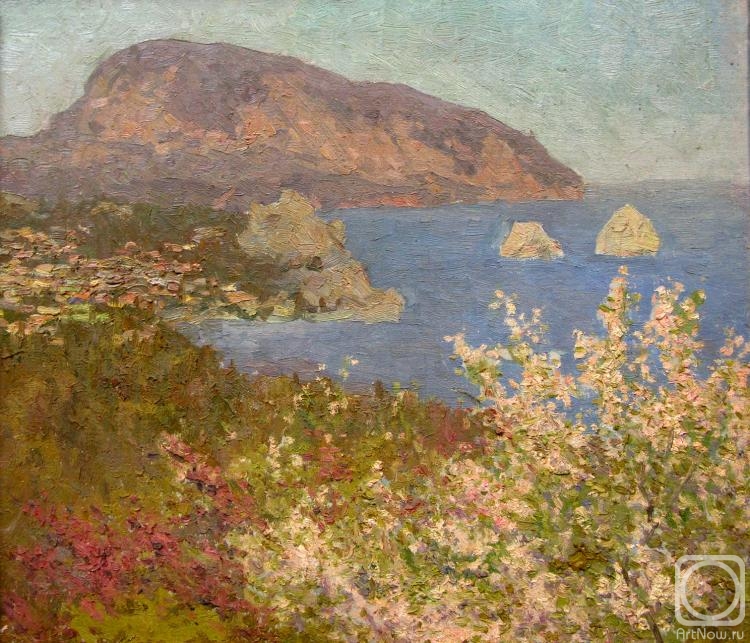This is an impressionist oil painting depicting a serene coastal landscape. The artwork is vertically rectangular and rich with textured brush strokes, evident throughout the piece. At the top, the sky is rendered in a greenish-blue hue with patches of brown, evoking a twilight ambiance. On the left, a rugged brown mountain adorned with patches of green trees and wildflowers, including cream, red, and white blossoms, slopes gently towards the water. The right side is dominated by a blue body of water, punctuated by several light brown rocks jutting from its surface, adding to the natural ruggedness. The foreground features vibrant green grass interspersed with various wildflowers, enhancing the painting's lush appearance. In the bottom right corner, there is an Instagram logo with the URL "artnow.ru," subtly incorporated into the artwork.